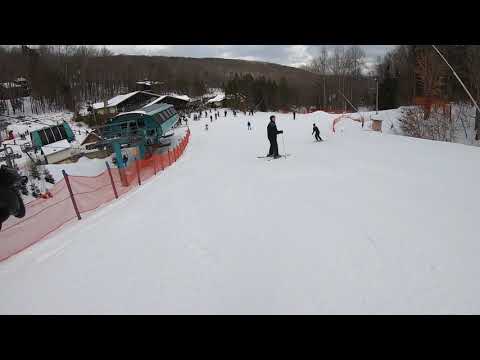The photograph depicts a bustling ski slope covered in fluffy white snow, framed in black. The scene primarily features a broad ski run that extends downhill from left to right, curving slightly to the right. In the foreground, on the right side, stands a skier dressed in all black, while another skier can be seen crouched, making their way downhill. The image also shows a well-populated area near the bottom left of the frame, where many skiers are gathered around a chairlift boarding station. An orange caution fence lines the left edge of the slope, sectioning off the area where an array of old buildings and two snow cats with side windows can be seen. Behind the chairlift, a lodge is visible. The landscape is adorned with leafless trees, and in the background, a mountain covered in dense forest rises majestically. A turquoise gondola with white accents ascends the mountain on the left. Despite the graininess of the photo, the lively activity on the slope and the natural beauty of the surroundings are evident.